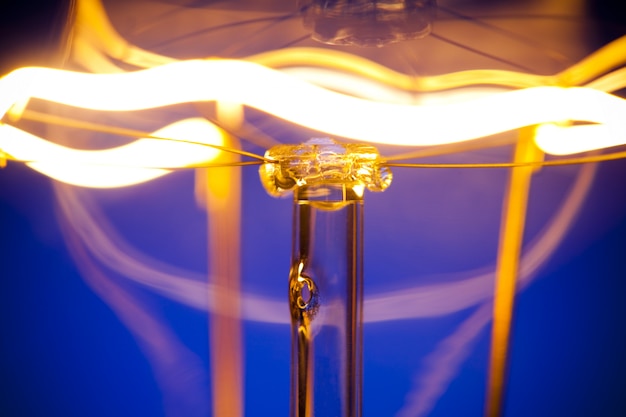This image captures a highly detailed close-up of the intricate inner workings of a light bulb against a blue, slightly blurred background. The photograph prominently features the filament, which is depicted as a bright yellow coil intertwined with a light white coil. Extending across the image, a thick white coil begins in the center, curves to the left edge, and then meanders back to the right, creating a sinuous, snake-like pattern. Supporting these coils is a clear glass stem with a small glass foundation that holds the wires delivering electricity. These fine, elongated wires span from one side of the image to the other, connecting the electrical arc essential for the light bulb's function. All these elements are sharply focused against the dim, reflective blue-black backdrop, which hints at the light bulb's overall silhouette.